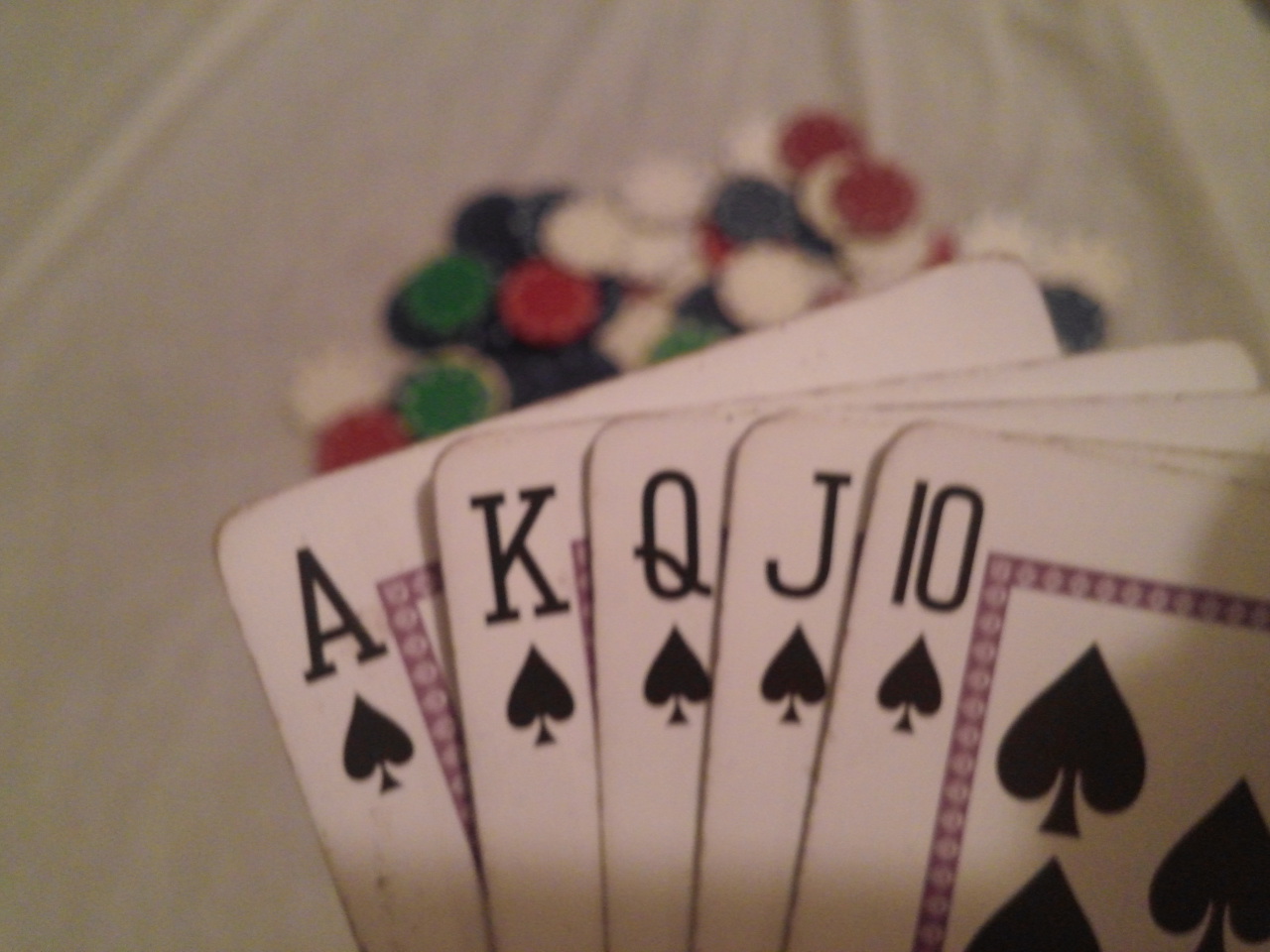This photograph captures a close-up scene from a poker game. In the bottom right corner, a scattered arrangement of playing cards is prominently displayed, albeit slightly soiled against the pristine white tablecloth backdrop. The cards are characterized by a noticeable reddish-brown border which accentuates their worn appearance. From right to left, the visible cards include the Ten of Spades, showcasing the number ten and a spade symbol beneath it, followed by the edge of a Jack of Spades peeking out slightly. Next in line is a Queen of Spades, fully exposed, with its distinctive "Q" and spade symbol, followed by the edge of a King of Spades. Finally, an Ace of Spades is evident on the far left, its red border partially visible. 

The table setting is further accentuated by a haphazard pile of poker chips at the center of the frame, comprising a mix of colors: white, red, green, and a deep, almost black-blue hue. These chips, likely in use during an ongoing game, contribute to the dynamic and engaging nature of this image, composed over a white tablecloth that has been bunched up in several places, adding texture and depth to the overall scene.